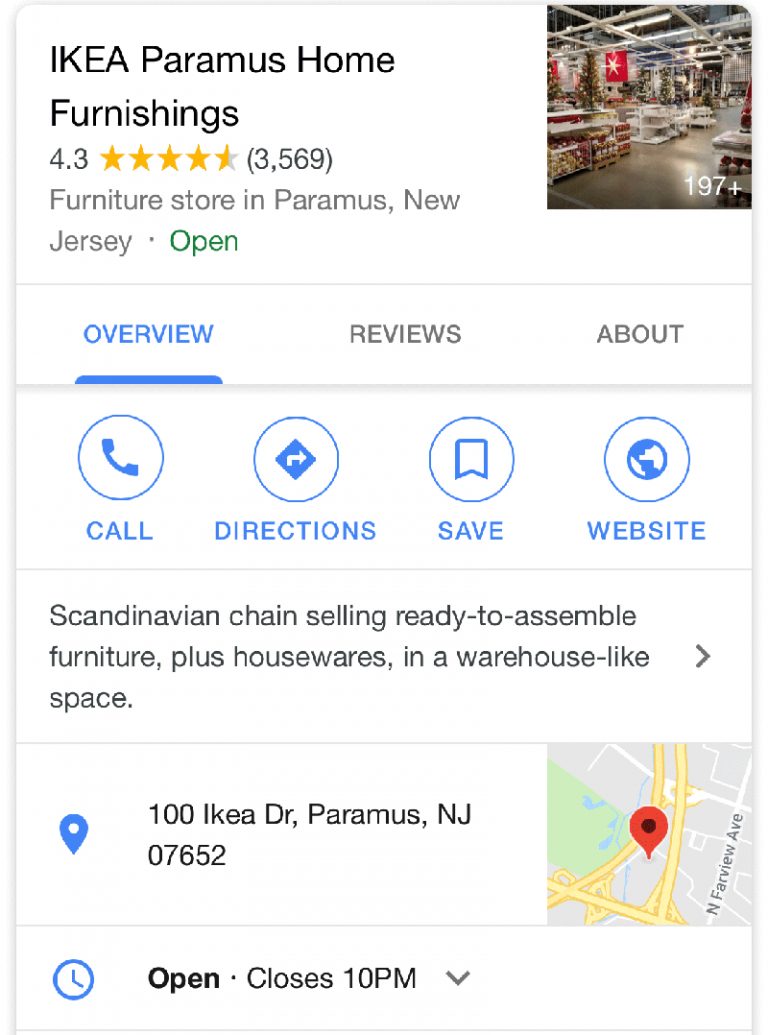**Descriptive Caption:**

A detailed Google Maps screenshot featuring the Ikea Paramount Home Furnishings store in Paramus, New Jersey. The webpage header prominently displays the store's name, Ikea, alongside its address and operational status—marked as open. A small image on the right showcases festive Christmas items, including Christmas trees and bulbs, listed at $197. The store boasts a 4.3-star rating from 3,569 reviews. 

Navigation options are clearly laid out with blue and white icons: 'Call', 'Directions', 'Save', and 'Website'. The 'Overview' tab is highlighted in blue, offering a concise description of the store, defining it as a Scandinavian chain specializing in ready-to-assemble furniture and housewares, housed in a warehouse-like space. The store's location is specified as 100 Ikea Drive, Paramus, New Jersey, 07652. An icon of a clock indicates the current opening hours, with the store closing at 10 p.m.